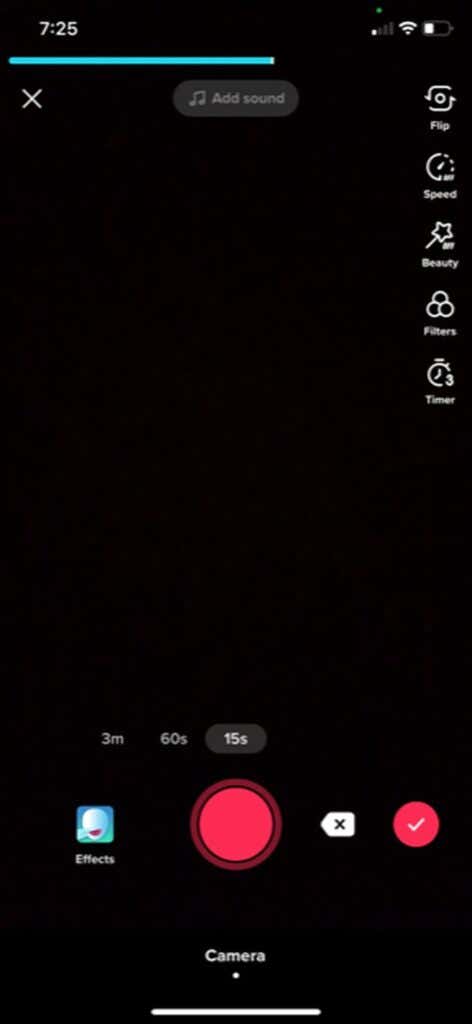This image is a screenshot from a smartphone, characterized by a pitch-black background. In the top left corner, white text displays the time, either "7:25" or "725". To the right corner, there's a battery icon showing about 30% charge (indicated by the white portion) and 70% remaining empty (black). Adjacent to the battery icon, there's a full Wi-Fi signal and partially connected internet signal where the first bar is white while the rest are gray.

Below the time display, a blue line extends slightly more than halfway across the screen, with a white "X" beneath it. Centered on the screen is a gray tab featuring a light gray music note and the words "Add sound". To its right, there's a camera icon labeled "Flip". Nearby, there is half of a circle on the left side with small dots down the right side, with the label "Speed". Below this, there's a wand symbol, angled upwards to the right, accompanied by the label "Beauty". Further down, two white-outlined circles are situated beside each other with a third on top, underlined with "Filters". A stopwatch icon follows, with a small "3" in the bottom right corner, denoted as "Timer".

The lower portion of the screen remains black until roughly two inches from the bottom where, about an inch from the left border, it reads "3M". Adjacent to this, a space is labeled "60S", followed by a gray tab inscribed with "15S" in white text. Beneath the "3M" designation lies a blue square featuring a white face with a pink mouth and the text "Effects". To the right, a prominent red circle with a red border exists, flanked on its left by a white square containing a black "X" and on its right by a red circle with a white check mark. Below the large red button, the word "Camera" appears, followed by a small dot and a line. At the screen's very bottom, a white line stretches horizontally, positioned about an inch from both the left and right edges.